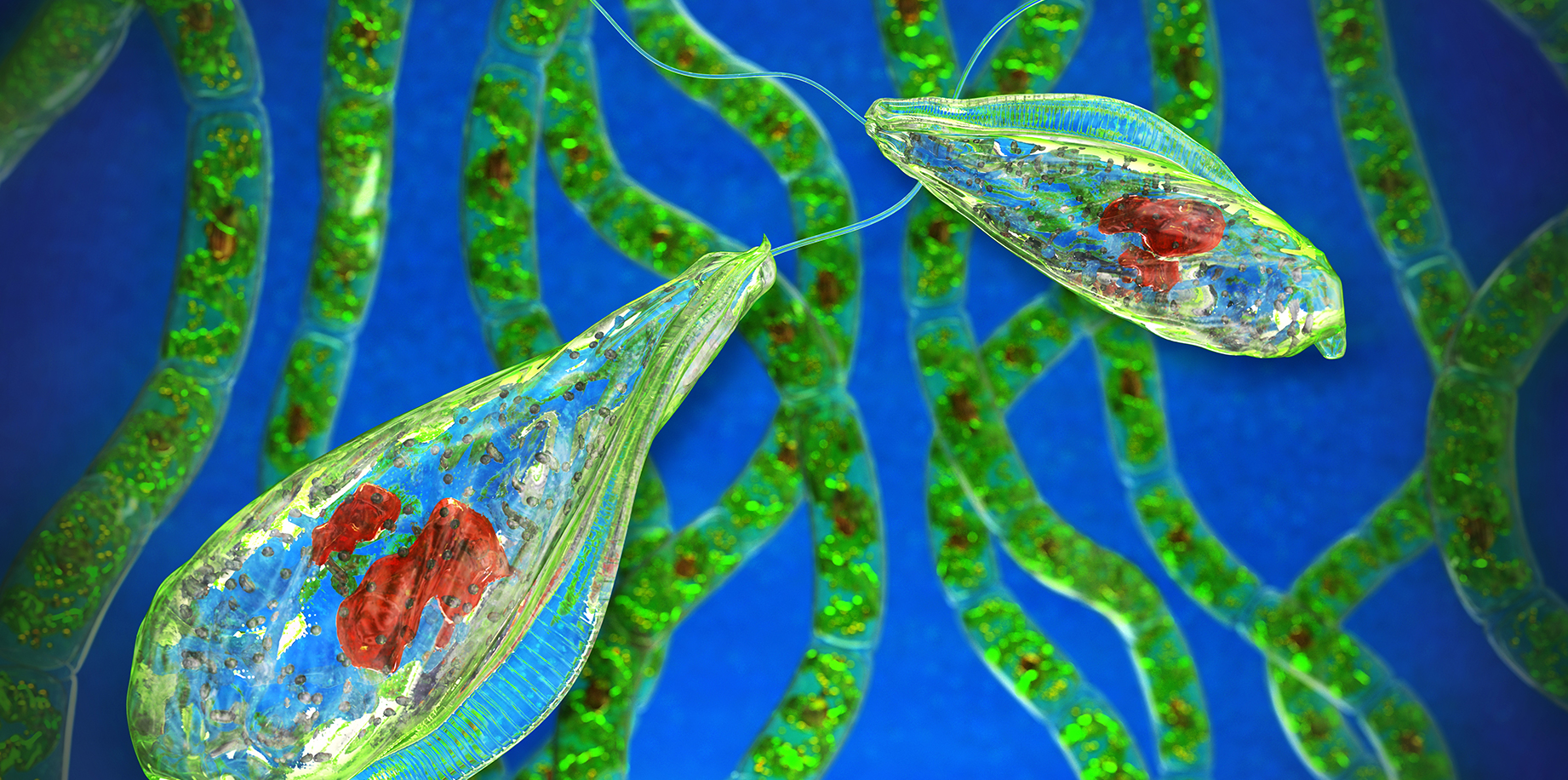The image depicts a highly detailed, computer-generated 3D illustration of two translucent, almost glass-like cells, likely of human, animal, or plant origin. Each of these cells contains a red, bean-like substance and a leafy green-brownish matter. The cells are clear and emit a white string-like tail at their ends. Set against an electric blue, slightly grainy background, the scene includes several long, wavy tubular structures segmented in shades of green, dark brown, and black, with occasional light and dark green spots, resembling an underwater environment. Additionally, curved, segmented bands of gold and orange with a grainy texture are also present in the background. The overall intricate illustration suggests a microscopic view, highlighting the detailed complexity of cellular structures and their surroundings.